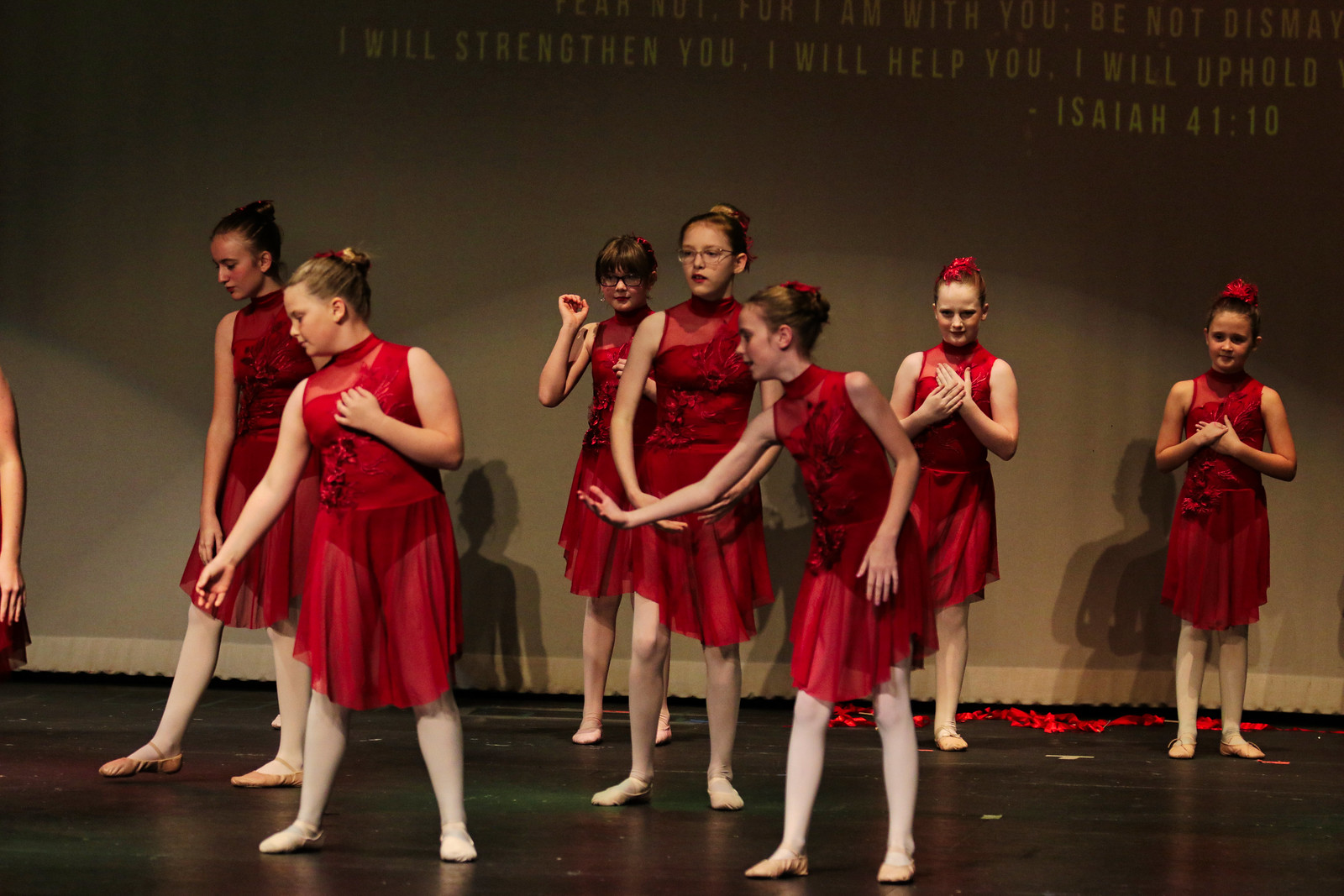This image captures an indoor stage set for a performance featuring a group of seven young girls dressed uniformly in red knee-length dresses. The stage floor appears to be a dark, possibly hardwood surface. The girls are arranged with two on the left, three in the center, and two on the right, each striking a specific pose. One girl on the left is looking left with her hand up in front of her chest, while another beside her has her feet pointed left with her right arm down by her side. The central figure faces slightly forward with her head turned left, her right arm extended in front of her, and a third girl directly behind her, wearing glasses, looks straight ahead. Two girls in the back near the right edge of the image face forward with their hands in front of their chests, sporting red ribbons in their hair. The backdrop features a large brown poster adorned with yellow text, partially cut off, but visibly quoting Isaiah 41:10, "I will strengthen you, I will help you, I will uphold..." The setting suggests the scene is part of a dance recital or rehearsal.